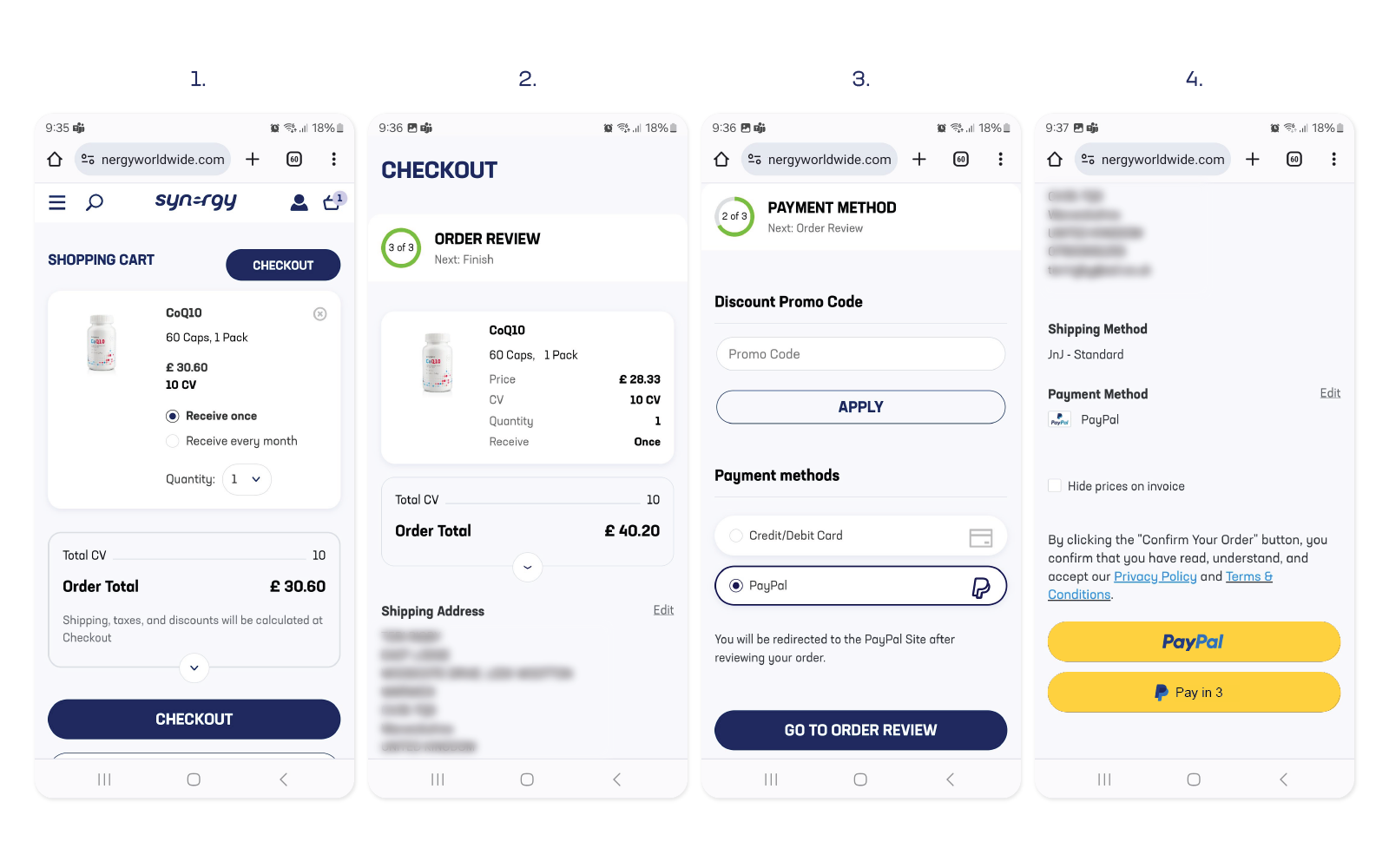This image is a detailed composite of four sequential screenshots taken from a cell phone, displaying the checkout process of an online purchase on a site called Synergy. Each screenshot is numbered sequentially from one to four, moving from left to right. 

1. **Screenshot One:** The first screenshot displays the typical cell phone status icons at the top, including carrier signal, battery percentage, and others. Below, it features a web page for Synergy (denoted as "S-Y-N" with a small "R-G-Y"). On this page, the shopping cart icon shows a single item, a capsule, with a total of £30.60. At the bottom, a prominent button labeled "Checkout" invites the user to proceed to the next step.

2. **Screenshot Two:** This screenshot is set against a gray background with the word "Checkout" in large bold letters at the top. Below this, the page indicates the user's current stage in the checkout process with a white block and a green circle. It shows "Order Review" in navy blue lettering beside it. The same information from the first screenshot is repeated here, but with added shipping costs, bringing the total to £40.20. The shipping address is displayed but has been blurred for privacy.

3. **Screenshot Three:** The third screenshot illustrates step two of the checkout process, focusing on the payment method. It includes a section for entering a discount promo code and an "Apply" button. Below that, there are options for payment methods, with PayPal highlighted as the chosen method. At the bottom of the screen, there is a "Go to Order Review" button in white text against a navy background.

4. **Screenshot Four:** The final screenshot reviews the order. The shipping address is again blurred, and it confirms the standard shipping method and PayPal as the payment method. A disclaimer states that by clicking "Confirm My Order," the user agrees to the terms and conditions. Below this, there are two yellow buttons: the first shows "PayPal" in its distinctive dark blue and light blue logo, and the second features the PayPal "P" logo with "Pay in 3" written beside it, indicating an option to split the payment into three installments.

This series of screenshots thoroughly details each step of the checkout process on the Synergy site, from viewing the shopping cart to confirming the order.